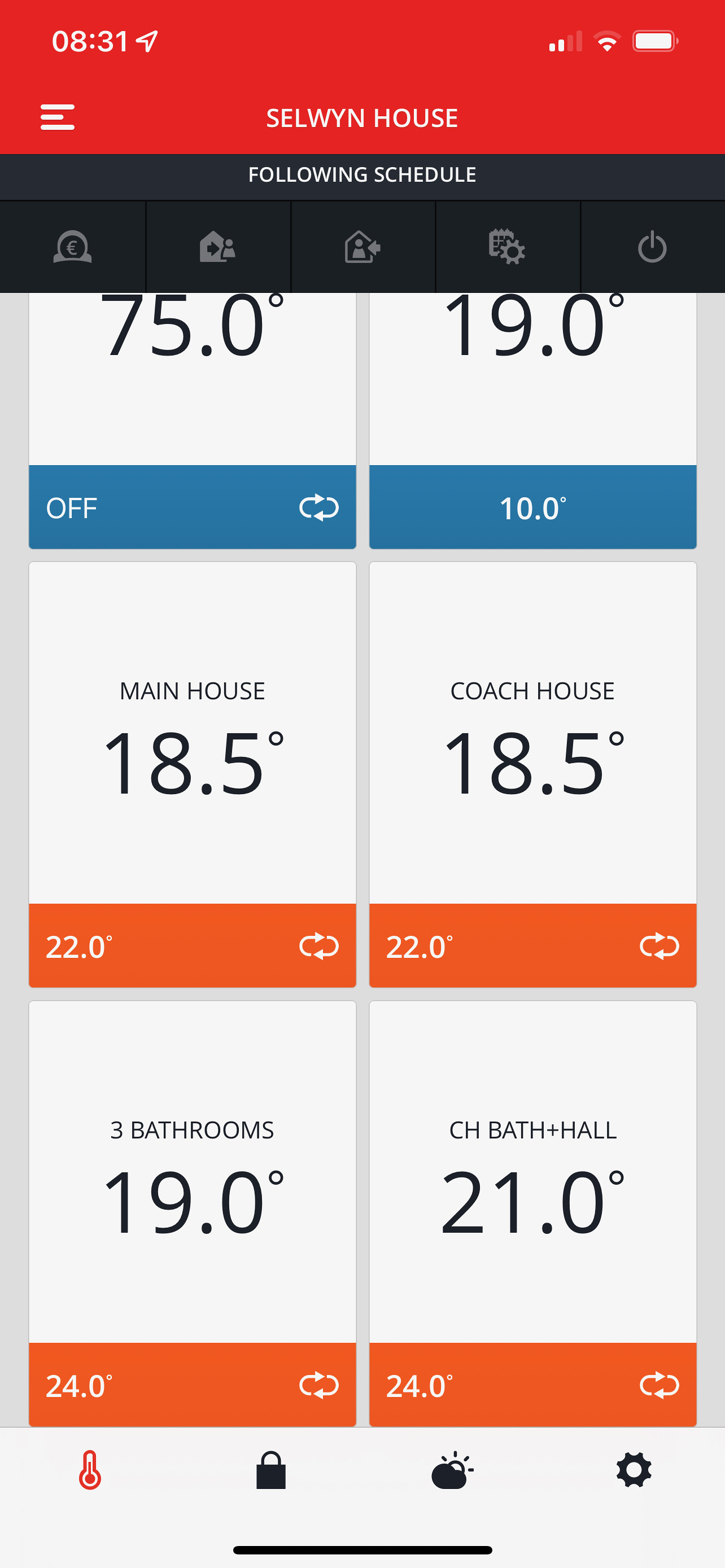This is a detailed screenshot captured from a mobile phone displaying a smart home application interface. Starting at the top, there is a prominent red status bar. On this red bar, the time is displayed as 8:31 in white font, accompanied by a location arrow icon indicating GPS is active. In the upper right corner of the red bar, there are icons showing a Wi-Fi signal at two bars, mobile data reception, and a fully charged battery.

Directly below the red status bar, the text "Cell Wynhouse" (S-E-L-W-Y-N house) is presented, followed by a navy blue bar with the phrase "Following schedule" in white font. Below this, the smart home application interface becomes visible, though the specific app name is not disclosed. There is a blue navigation bar with multiple icons allowing further exploration of the app.

The main content area of the screen features six "smart home cards," each representing different zones of the home along with their respective temperatures and statuses. The first card, partially cut off, shows a temperature of 75°F and is marked "off." The second card, also slightly obscured, lists a temperature of 19.0°C and a status of "10."

Continuing downward, four more smart home cards are clearly visible:
1. Main House: 18.5°C
2. Coach House: 18.5°C
3. Three Bathrooms: 19.0°C
4. Hall and Bath: 21.0°C

Each of these cards provides specific temperature readings for different areas, giving a comprehensive overview of the home's climate control settings.